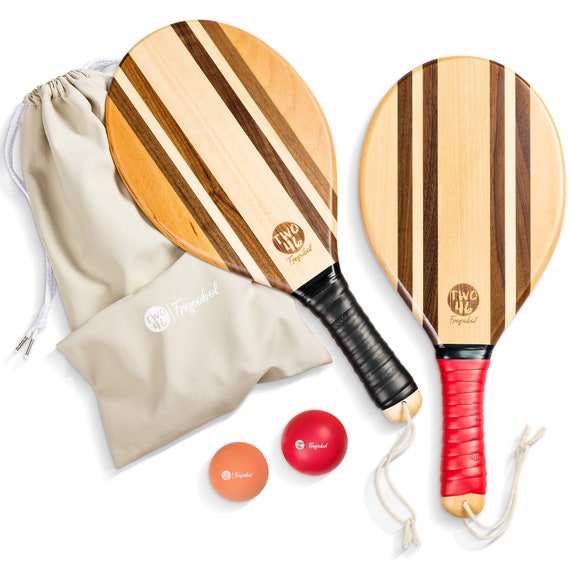The image displays two light-colored wooden ping pong paddles with dark vertical stripes lying flat on a solid white surface. Each paddle features a white logo near the handle, with the number "246" and brown circle logos. The paddle on the right has a red leather handle, while the one on the left has a black leather handle, both with strings tied to them. Positioned at the bottom center of the image are two balls, one red and the other peach-colored, each adorned with white logos. To the left, there's a beige cloth pouch with a white logo lying underneath the left paddle.